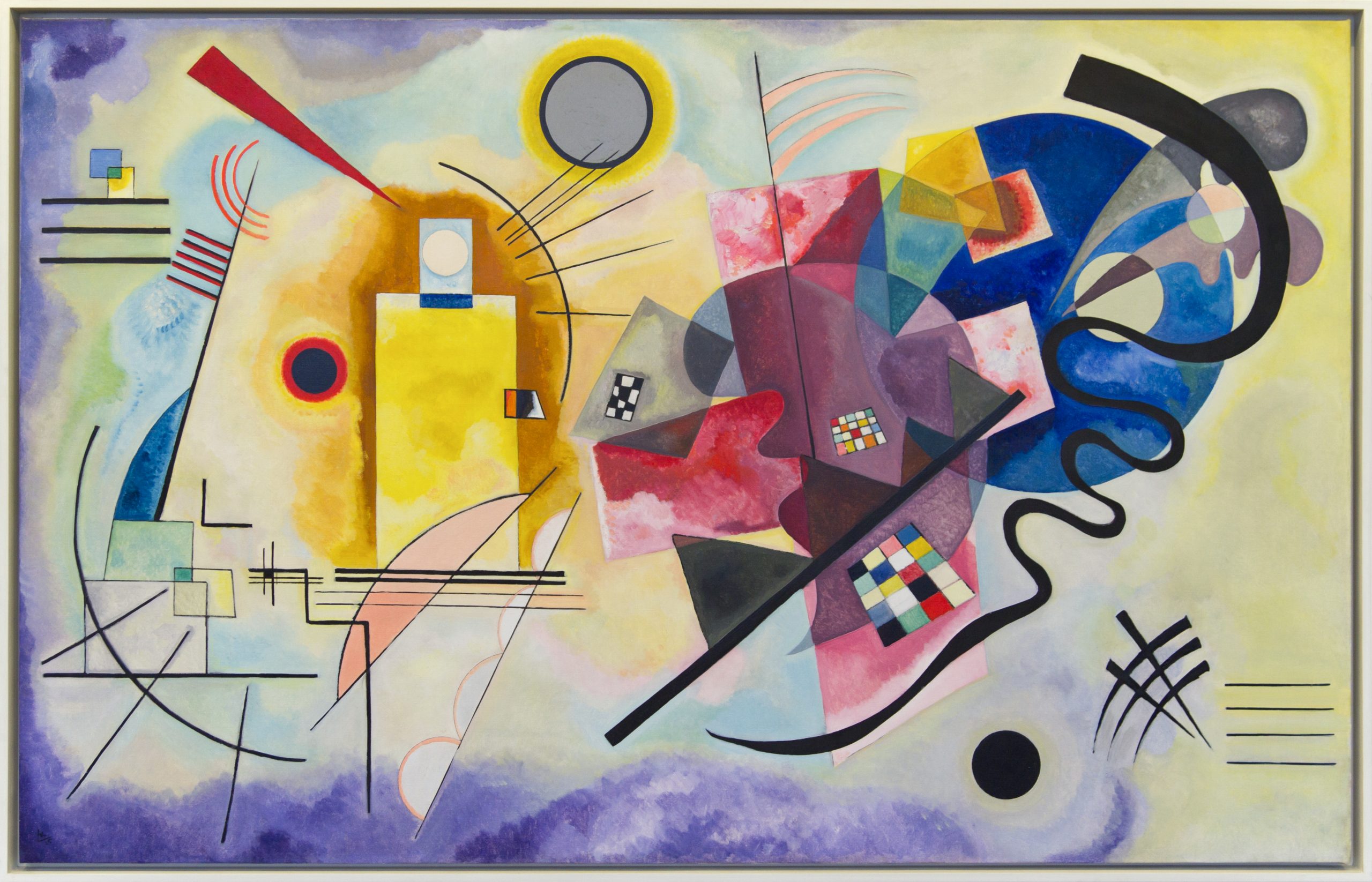This modern painting, reminiscent of cubist and abstract styles, intricately blends stark geometries with soft pastel washes. Dominating the left side, a yellow humanoid-like head emerges, composed of a yellow rectangle, several curved lines, and a red triangle. Prominently, a red circle with a black dot inside, resembling an eye, enhances its complexity. As we move rightward, chaos and abstraction intensify with interlocking shapes: a blue circle, a purple half-circle, and black squiggly lines. Amidst these, checkerboard patterns intermittently appear, varying from black and white to multicolored grids. The background interweaves subtle hues of yellow, blue, and purple, akin to watercolors, contrasting with the bold black lines and curves that overlay it. In the bottom right corner, striking black dots, horizontal lines, and intersecting diagonal lines add to the dynamic complexity of the painting, leaving its interpretation open to the viewer's imagination.